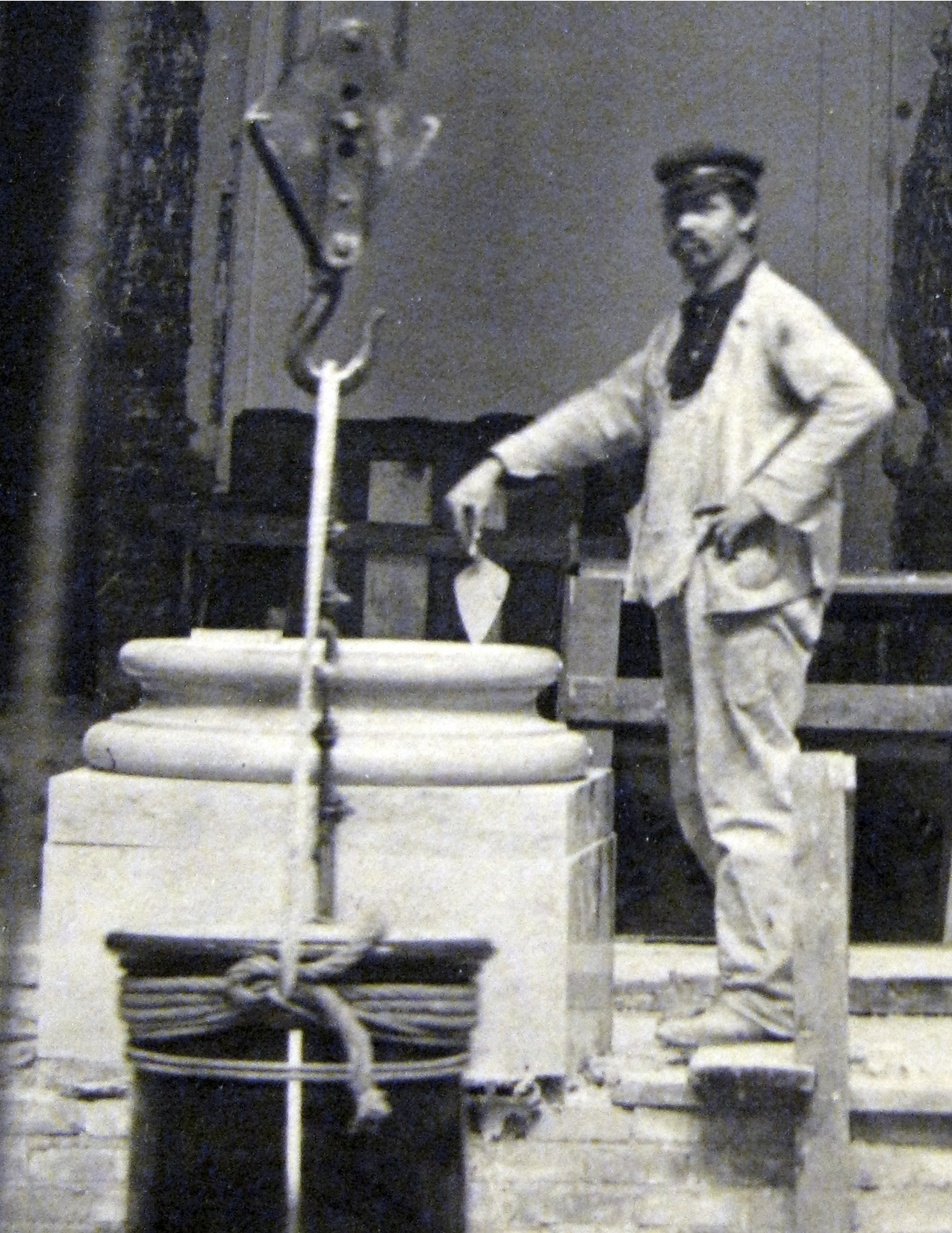This black and white vintage photograph, possibly from the 1940s or 1950s, features an industrial or construction scene. A man stands on a wooden plank, next to a large pot or basin suspended by ropes from a metal hook, likely connected to a crane overhead. He is dressed in a long-sleeve white coverall jacket over a dark shirt, accompanied by baggy trousers. He dons a dark driver's cap or possibly a bandana, and sports a large mustache. In his hand, he holds a trowel or scraper tool, suggesting that he is engaged in some form of labor or construction work. The overall industrial setting, combined with the man's attire and the equipment around him, paints a vivid picture of mid-20th-century manual labor.